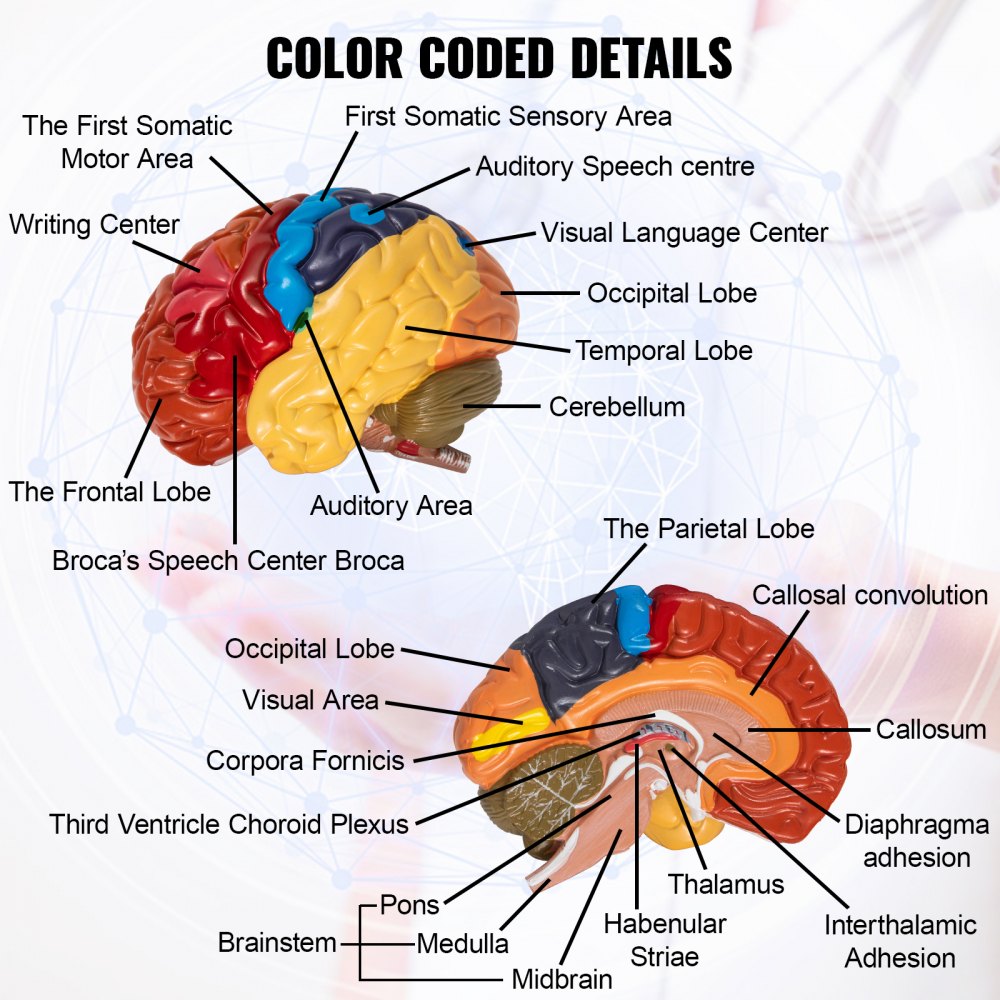This diagram illustrates a human brain with color-coded details. The title at the top reads "Color-Coded Details" in black text. The top-left section of the diagram displays a side view of the brain, with each region colored differently—red, blue, dark blue, yellow, orange, and brown. Black arrows point to various parts, highlighting specific areas such as the first somatic sensory area, first somatic motor area, writing center, frontal lobe, temporal lobe, occipital lobe, visual language center, auditory speech center, and the Broca speech and auditory areas. The bottom-right section of the diagram shows a sagittal view of the brain, sliced down the middle to reveal internal structures. This section is also color-coded, with black arrows indicating regions like the colossus, thalamus, midbrain (colored pink), pons, corpus callosum, visual area, and parietal lobe (colored dark navy blue).